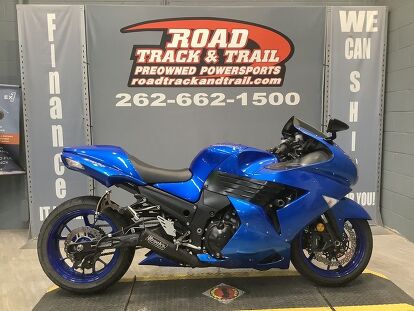This photograph captures a sleek, royal blue sport motorcycle, positioned indoors on a tan tiled floor, likely within a showroom. The motorcycle, which is facing to the right, appears shiny and new, featuring a bright cobalt blue body and chassis, accented by a black leather saddle seat. Additional cobalt blue elements include the seat hump at the front and a tailpiece behind the seat. The motorcycle is equipped with black tires and black spokes centered around dark gray hubs, along with a black, slightly rising windscreen, black handlebars, and a black rearview mirror.

Behind the motorcycle, a gray wall serves as a backdrop. Prominently displayed on this backdrop is a logo featuring a red swoosh outlined in black, curving to the left. Superimposed on the swoosh is the text "ROAD TRACK AND TRAIL" in bold white capital letters. Below this, smaller white printed text reads "PRE-OWNED POWER SPORTS," and directly beneath it, slightly smaller italicized bold white text states "ROADTRACKANDTRAIL.COM." A larger bold white phone number, "262-662-1500," is listed at the bottom of the logo. Additionally, the left side of the backdrop has vertical text reading "FINANCE" in bold white letters, while the right side features two lines of horizontal text stating "WE" and "CAN," followed by partially obscured vertical text. The entire setup and design convey a professional, marketing-oriented presentation aimed at showcasing the motorcycle for potential buyers.